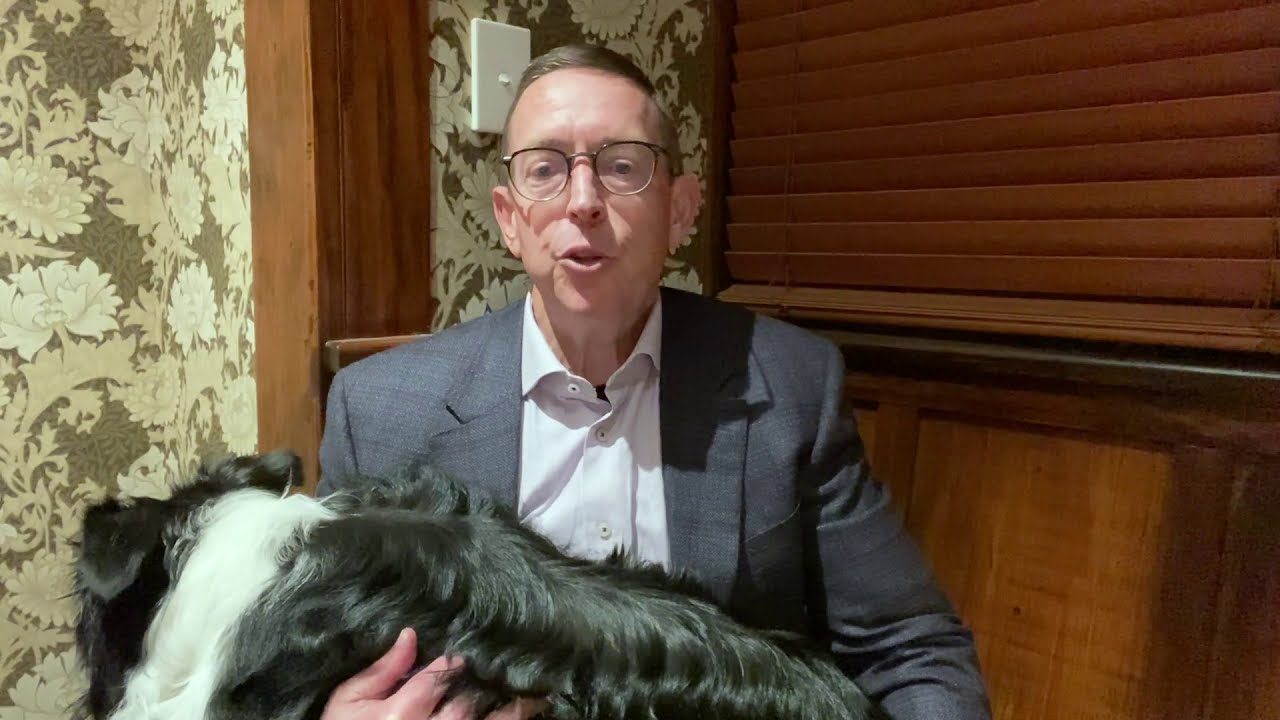In this detailed image, we see a Caucasian man with neatly cut, thinning brown hair and a high forehead, giving a narrow, oval-shaped appearance to his face. He wears black-rimmed glasses and a gray suit jacket over a white button-down shirt, unbuttoned at the top. The man is seated, holding a furry black-and-white dog, which faces away from the camera, showing off its black coat with a white patch around its neck, possibly a border collie. He is in the midst of speaking, with shadows cast on his face from unseeable lighting. The background features a wall with a soft olive green, beige, and brown leaf-patterned wallpaper on the left side, partially divided by a wooden board that runs vertically. On the right, wooden horizontal blinds cover a window, and a wooden booth or chair is visible. A white light switch is mounted on the wall, and the setting overall suggests a warm and inviting indoor environment.